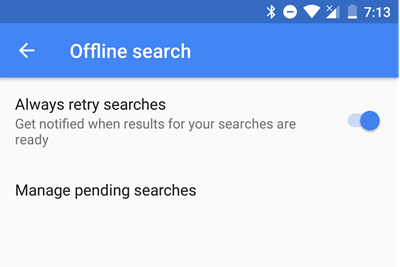This image is a screenshot from a smartphone, showcasing various interface elements. 

At the very top, there is a dark blue status bar. The left side is blank, while the right side features several icons in white: the Bluetooth logo, a "Do Not Disturb" symbol (circle with a line through it), the Wi-Fi logo, and a signal strength indicator represented by bars in a triangle shape with an "X" on top. Following these is a battery icon showing approximately 20% battery life remaining. The time displayed is 7:13.

Directly below the status bar is a slightly lighter blue banner. On the left side of this banner, there is a left-pointing arrow, next to which is the text "Offline Search."

Beneath this banner is a gray background area. It starts with the text "Always retry searches" in a bold black font. Below this, in a darker gray font, it says "Get notified when results for your searches are ready." Next to this text is a toggle switch, which is set to the right, indicating that the feature is turned on. 

Further down, it reads "manage pending searches," suggesting a link or option related to search management.